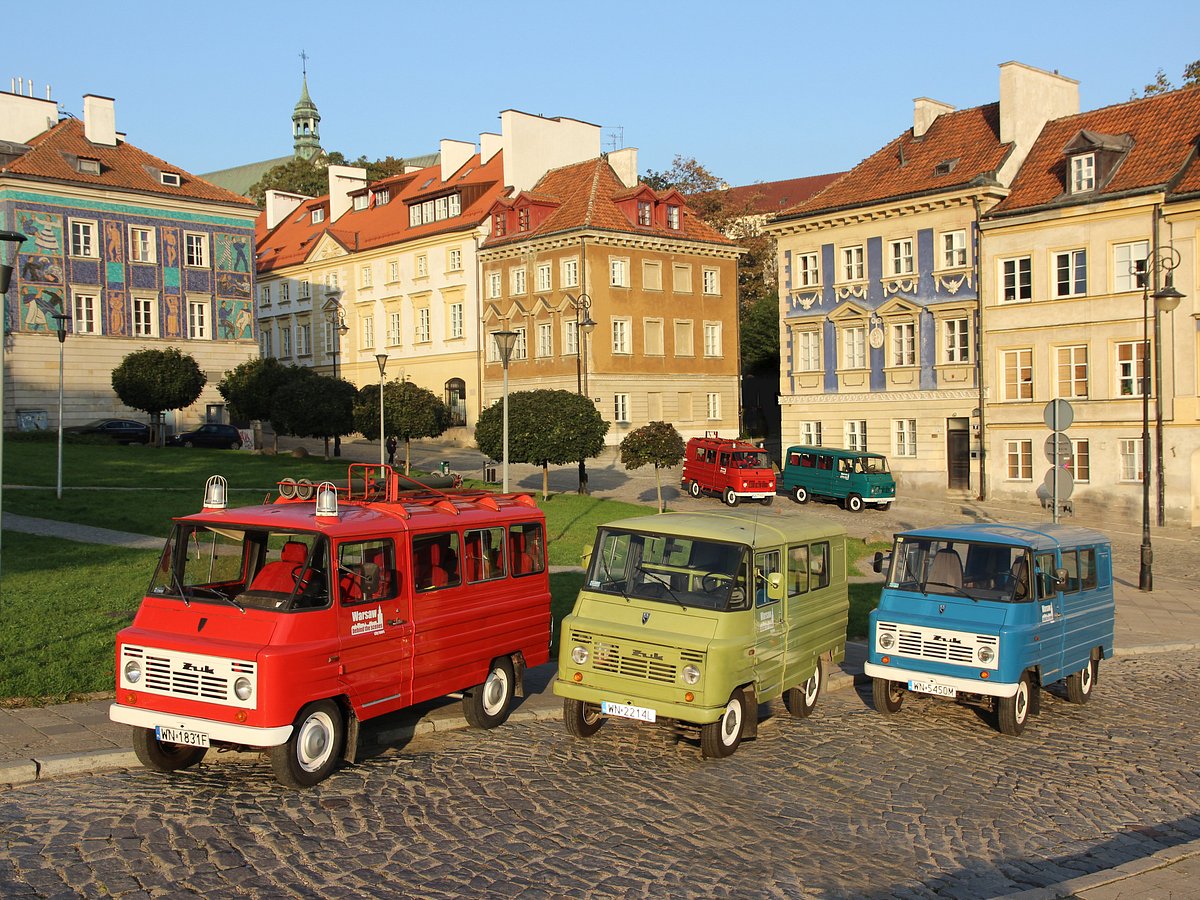The photograph depicts a scene in what appears to be an old, possibly Eastern European city, characterized by stone-covered buildings, some painted in blue and brick colors with one on the far left adorned with mosaic tiles. In the foreground, a cobblestone road runs from the bottom left corner to the right, lined with three old vans facing left. The van on the left is red with additional features such as two lights and some handle-like structures on the top, suggesting it might be an emergency vehicle. The middle van, which is slightly elevated, is a lime green color, and the one on the right is blue. Intriguingly, the scene includes green space with wide, oval-shaped tree leaves and scattered street lamps. The background showcases a row of two to three-story buildings with light brown facades and varying shades of angled, brown rooftops dotted with chimneys. Additionally, two more vehicles—a red van and a dark green van—are parked near the buildings, emphasizing the blend of historical architecture and dated vehicles against a clear blue sky. Despite some elements appearing slightly surreal, the image blends modern and vintage aesthetics, providing a glimpse into a picturesque urban setting.